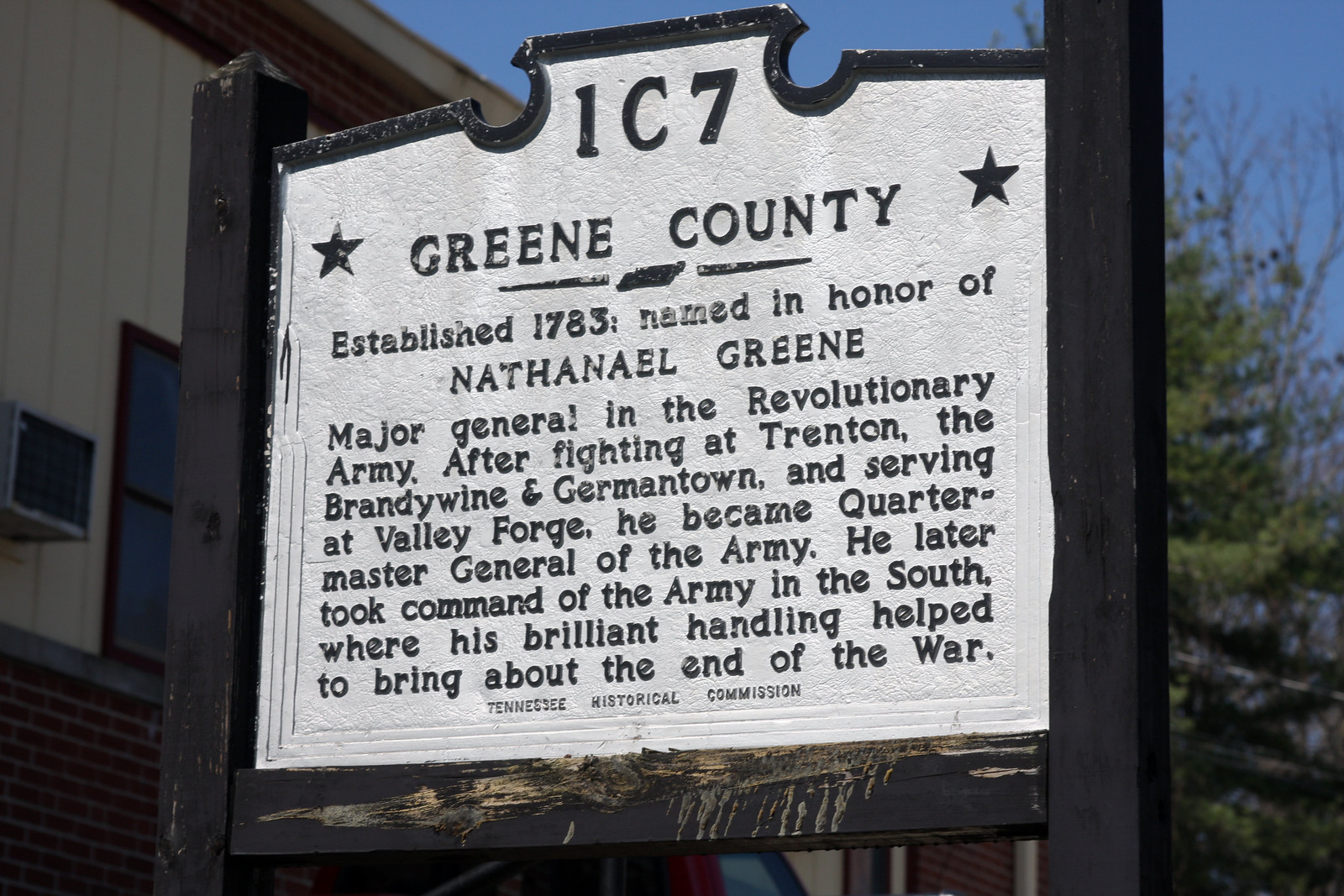This is an outdoor image of an old wooden historical marker with black posts and a black border. At the top of the white sign is the number IC7 and an image of the state of Tennessee, flanked by two stars. The sign commemorates Greene County, established in 1783, and named in honor of Major General Nathaniel Greene, a distinguished figure in the Revolutionary War. The text details Greene's contributions, mentioning his participation in pivotal battles such as Trenton, Brandywine, and Germantown, as well as his service at Valley Forge. It notes his role as Quartermaster General and his command in the South, which was instrumental in ending the war. At the bottom, in small capital letters, it reads "Tennessee Historical Commission." The bottom of the sign shows noticeable scraping and damage. In the background, there is a large building with an air conditioning unit, a tree, and a clear blue sky. The sign is supported by a wooden stand.